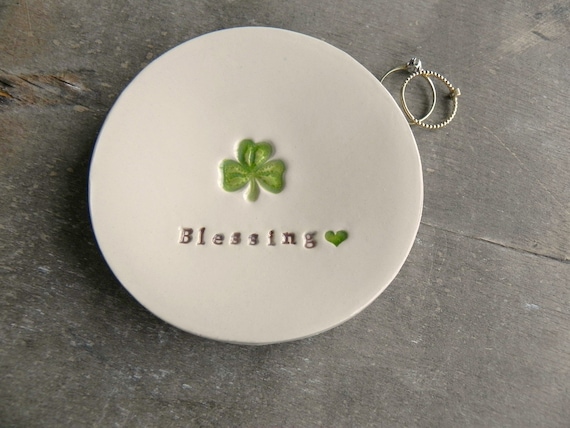The image is a detailed photograph of a small, circular white disc with a three-leaf clover design in the center, etched with a touch of white for detailing. Below the clover, the word "blessing" is etched in gray, accompanied by a green heart to the right. The disc is placed on a stone or concrete flooring. To the top right of the disc, lying on the same stone floor, are a pair of silver hoop earrings. Each earring features one small stone—one possibly a diamond, and the other perhaps an amethyst. The earrings are positioned so that one earring partially overlaps the other, yet both maintain contact with the stone surface beneath them.